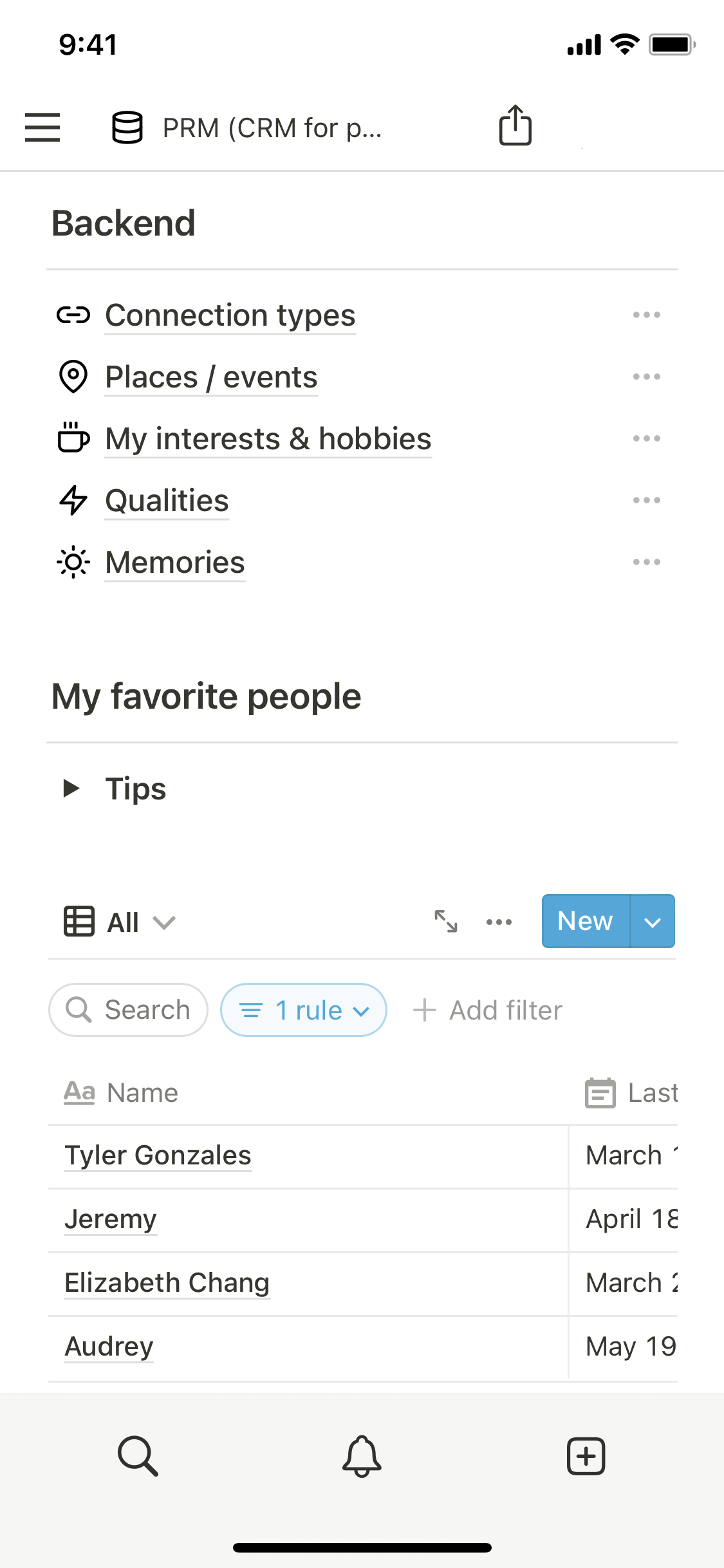This image appears to be a screenshot taken on a smartphone, likely an iPhone. The screen displays an application interface against a white background with various elements and text. The time on the phone reads 9:41 AM, and both the network signal strength and Wi-Fi signal are strong. The battery indicator suggests that the battery is fully charged or nearly so.

At the very top, on the upper left, there is a hamburger menu icon (three horizontal lines) next to the text "PRM" followed by "CRM4P" inside parentheses. A partial text follows, indicated by three trailing dots. An icon depicting three stacked disks, resembling a barrel, is also present, alongside a share button.

Below these elements, there is a header labeled "back-end" written as one word. Following this, several icons paired with labels are arranged vertically:
1. A linked chain with the text “Connection Types.”
2. A map marker icon labeled “Places/Events.”
3. A coffee cup emitting steam with the label “My Interests and Hobbies.”
4. A lightning bolt icon for “Qualities.”
5. A sun icon labeled “Memories.”

Each of these lines has an ellipsis (three dots) on the right-hand side, although their function is unclear.

Further down, a section titled "My Favorite People" appears. Adjacent to it is the word "Tips" with a black arrow pointing to the right. Below is a drop-down menu labeled "All," accompanied by an icon that looks like a small notebook page. Next to this drop-down menu are additional options: an ellipsis for more actions and a blue button labeled "New."

A small search box is visible, along with a label that reads "One rule" and another option to "Add a filter." It appears that a filter may have already been applied.

The list of names starts with:
1. Tyler Gonzalez (March).
2. Jeremy (April 1 or 18).
3. Elizabeth Chang (March).
4. Audrey (May 19).

The calendar icon next to each name suggests date entries, but the meaning of "last" adjacent to the calendar icon is obscured, possibly requiring horizontal scrolling to view fully.